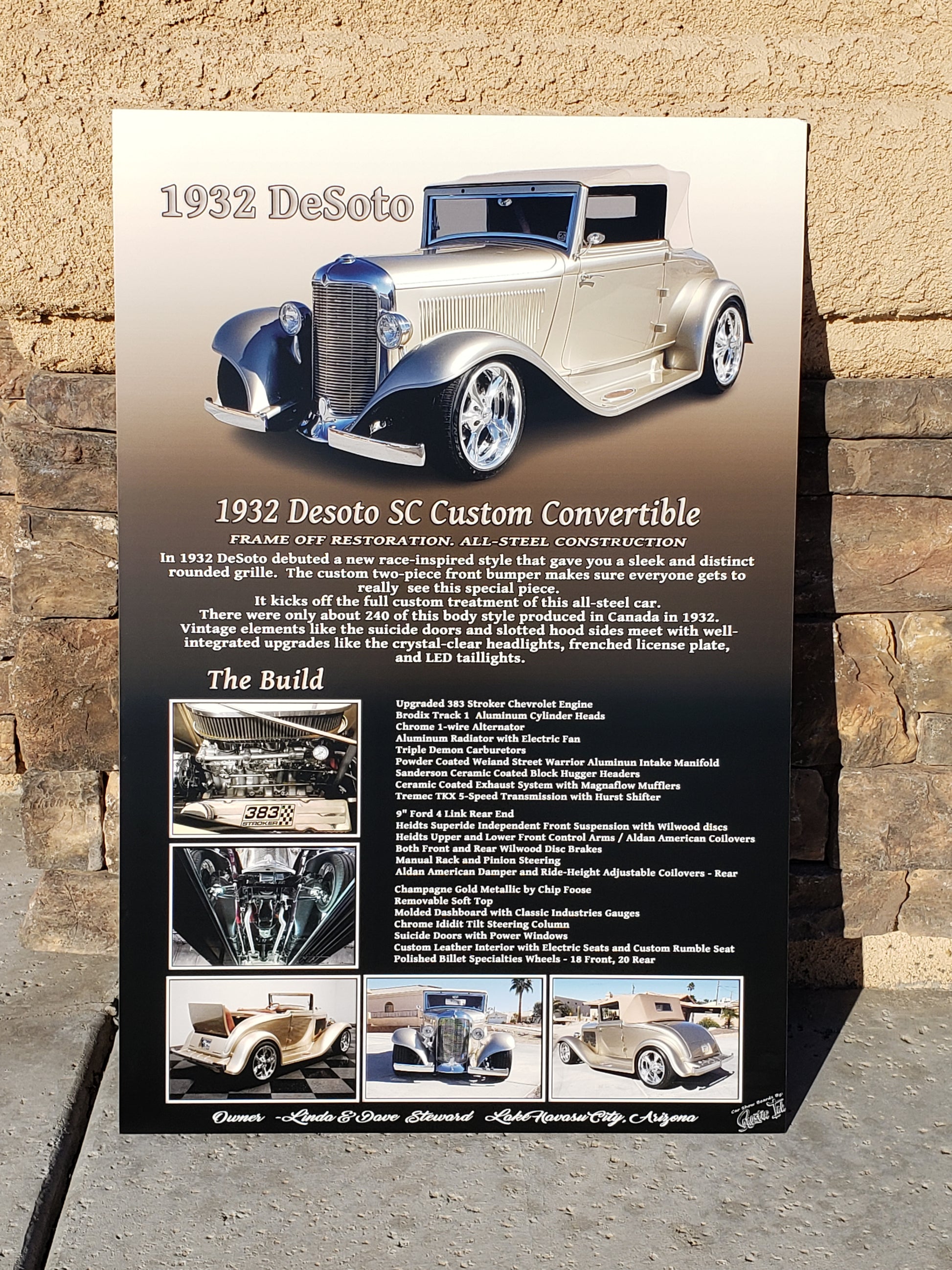This is a photograph of an advertisement poster for a 1932 DeSoto SC Custom Convertible Hot Rod, propped against a stone building on a concrete sidewalk. The banner prominently features a vintage silver-gray 1932 DeSoto car angled to show its left front. The car displays a sleek, chrome grille and a custom two-piece front bumper. Above the car, the text reads "1932 DeSoto" in silver lettering with a black outline, and below it, the text "1932 DeSoto SC Custom Convertible" is featured in white with a black outline. Detailed paragraphs below this highlight features such as "frame off restoration" and "all steel construction," emphasizing its race-inspired style and distinct rounded grill. Surrounding the main text are multiple photographs showcasing various angles of the vehicle, including the front, side, rear trunk, and interior engine compartment with a chrome engine marked "383." The overall background of the poster is predominantly black, bringing focus to the car and the descriptive text.